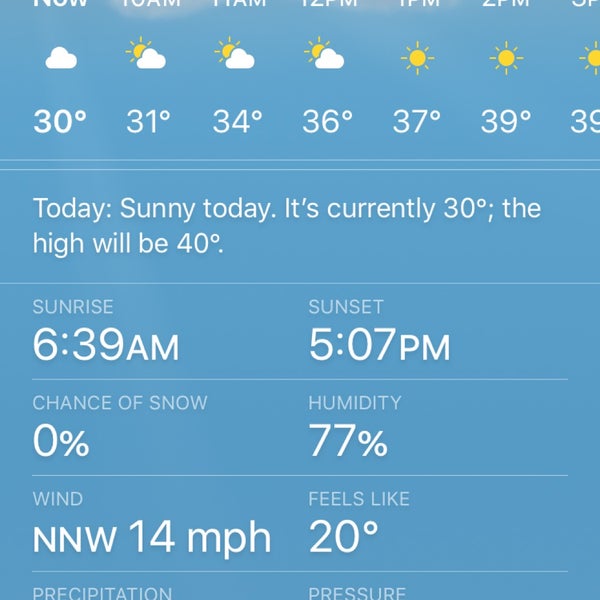This image features a screenshot of the Apple Weather app, with a light sky-blue background. At the top, the time information is partially visible, showing the hourly forecast starting from the left with "Now" followed by "10 AM," "11 AM," "12 PM," "1 PM," "2 PM," and "3 PM." Below these time labels, the temperatures per hour are displayed: 
- 30 degrees with a cloud icon for cloudy conditions 
- 31 degrees with both cloud and sun icons for partly cloudy 
- 34 degrees with similar icons 
- 36 degrees indicating partly sunny 
- 37 degrees and 39 degrees both show sunny conditions.

A section labeled "Today" states the current temperature of 30 degrees with a high of 40 degrees expected. The app also displays sunrise and sunset times, with sunrise at 6:39 AM and sunset at 5:07 PM. Following this, it indicates a 0% chance of snow, 77% humidity, and a northwest wind blowing at 14 mph. The "Feels Like" temperature is shown as 20 degrees.

The bottom part of the image contains two more labels, "Precipitation" and "Pressure," but the details are cut off and not visible in the screenshot.